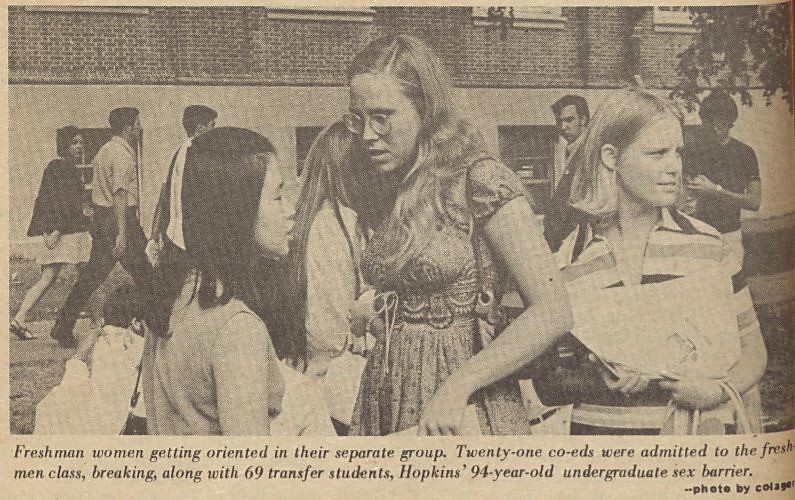This black and white newspaper clipping captures a historic moment at Hopkins University in the 1970s, marking the admission of female freshmen and transfer students, breaking the institution's 94-year-old undergraduate sex barrier. The central group in the image consists of three young women—two white and one Asian—engaged in conversation and orientation activities. One woman, dressed in a striped shirt, gazes into the distance, while another with glasses interacts with her peers. In the backdrop, additional students are seen walking near a brick academic building adorned with windows. The image, vintage in style, portrays a significant stride towards gender inclusion at the university.